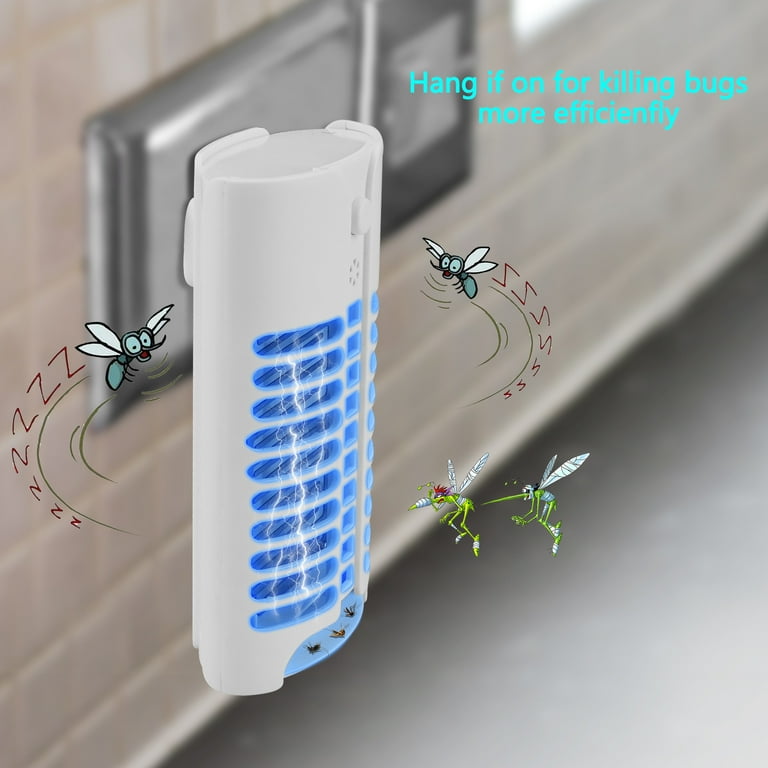In this commercial-like image, the central focus is a white, vertically elongated bug zapper plugged into a metallic outlet on a white brick wall. The device, resembling a long oval or rectangular container, features a plastic casing with multiple light blue, grill-like horizontal lines that are glowing blue, suggesting an electrified inner mechanism. Surrounding the zapper are cartoon illustrations of various bugs, including flies and mosquitoes, depicted in blue, green, yellow, and black colors, flapping their wings with 'zzzz' emanating from them. The background of the image is slightly blurred, with a grayish, metallic concrete floor. In the upper right corner, turquoise text reads, "Hang on for killing bugs more efficiently," though it appears to contain a typographical error. The image has a perfectly square format, contributing to its structured composition.